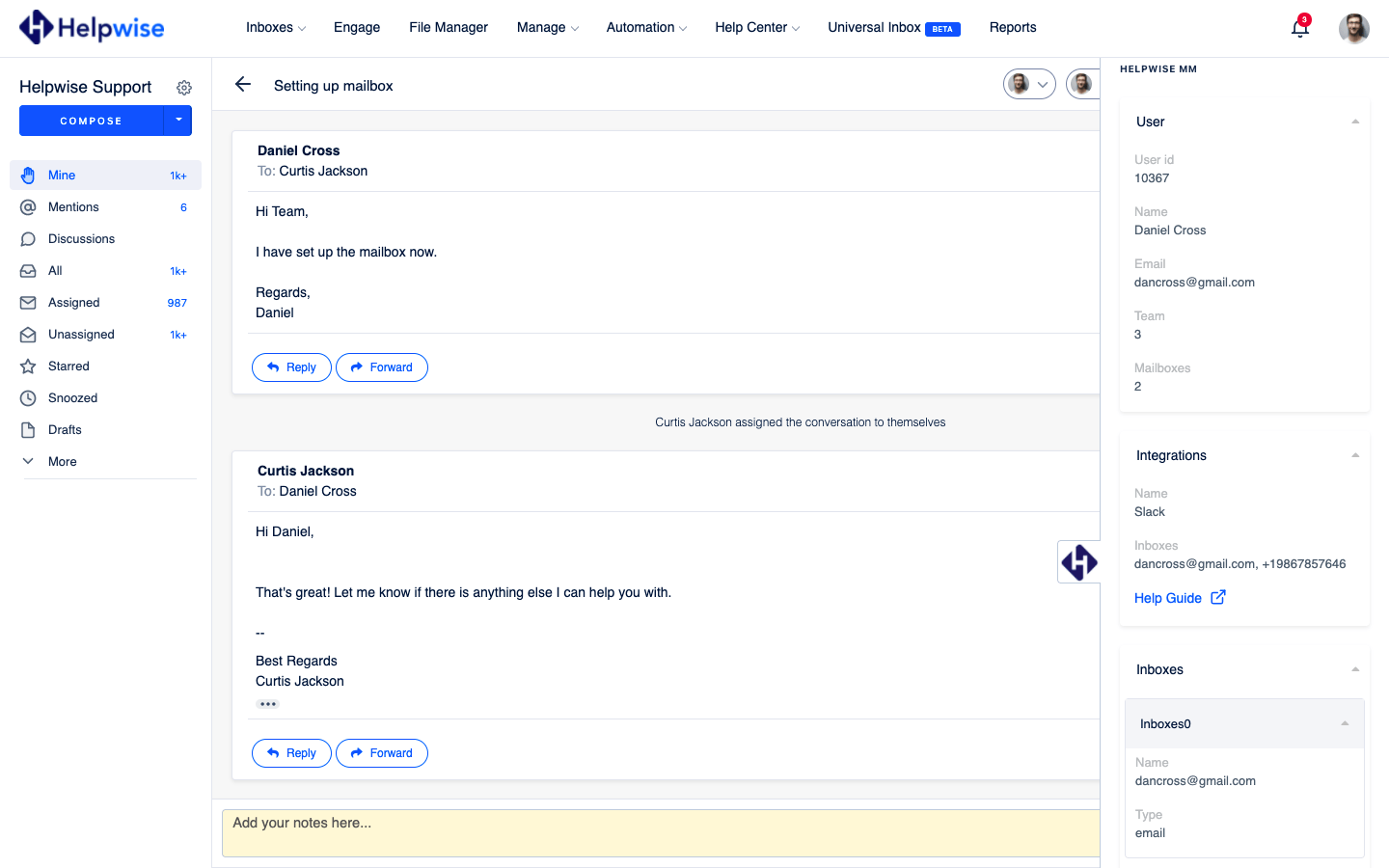A screenshot of the Helpwise website captures an organized layout with a functional dashboard on the left side of the screen. The dashboard begins with the section titled "Helpwise Support" and features a prominent "Compose" button for starting new messages. Below this, there are numerous sorting options such as "Mine," "Mentions," "Discussions," "All," "Assigned," "Unassigned," "Starred," "Snooze," "Drafts," and more. The "Mine" category lists over 1,000 messages, "Mentions" includes 6 messages, "All" also exceeds 1,000, "Assigned" contains 987, and "Unassigned" surpasses 1,000 messages.

In the center of the screen, a highlighted message from Daniel Cross to Curtis Jackson is displayed, reading: "Hi, team, I have set up the mailbox now. Regards, Daniel." Directly below this message, there are options to reply or forward. The subsequent message on the thread is Curtis Jackson's response to Daniel Cross, which states: "Hi, Daniel. That's great. Let me know if there is anything else I can help you with. Best regards, Curtis Jackson."